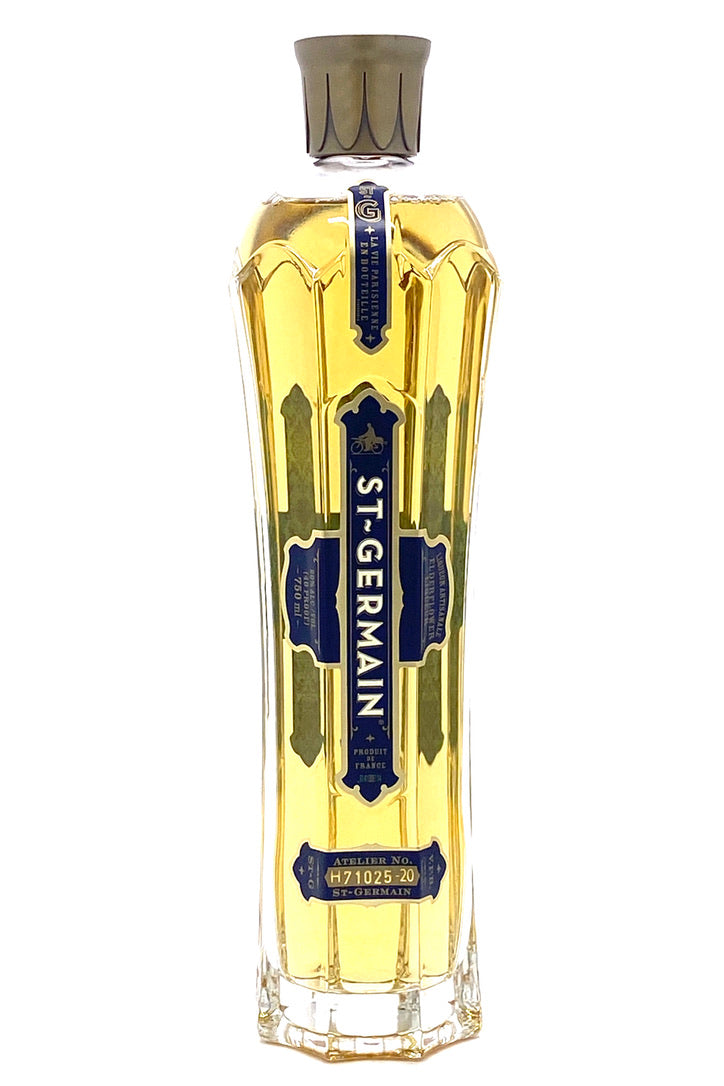The image features a towering, elegant bottle of Saint Germain liquor, distinguished by its clear, thick glass construction which reveals the yellowish, transparent liquid inside. The bottle boasts an elaborate, scalloped design extending from its sophisticated, solid gray cap down its vertical lines of glass. A prominent, minimalistic blue label with silver trim, shaped somewhat like a cross or a band with intricate details, runs vertically along the bottle, allowing the contents to be showcased. Additional delicate labeling at the base includes a serial number, Atelier H71025-20, affirming its exclusivity and high quality. The bottle also details its contents as Elderflower, 750 milliliters, and 70 proof, indicating a luxurious and finely crafted alcoholic beverage.